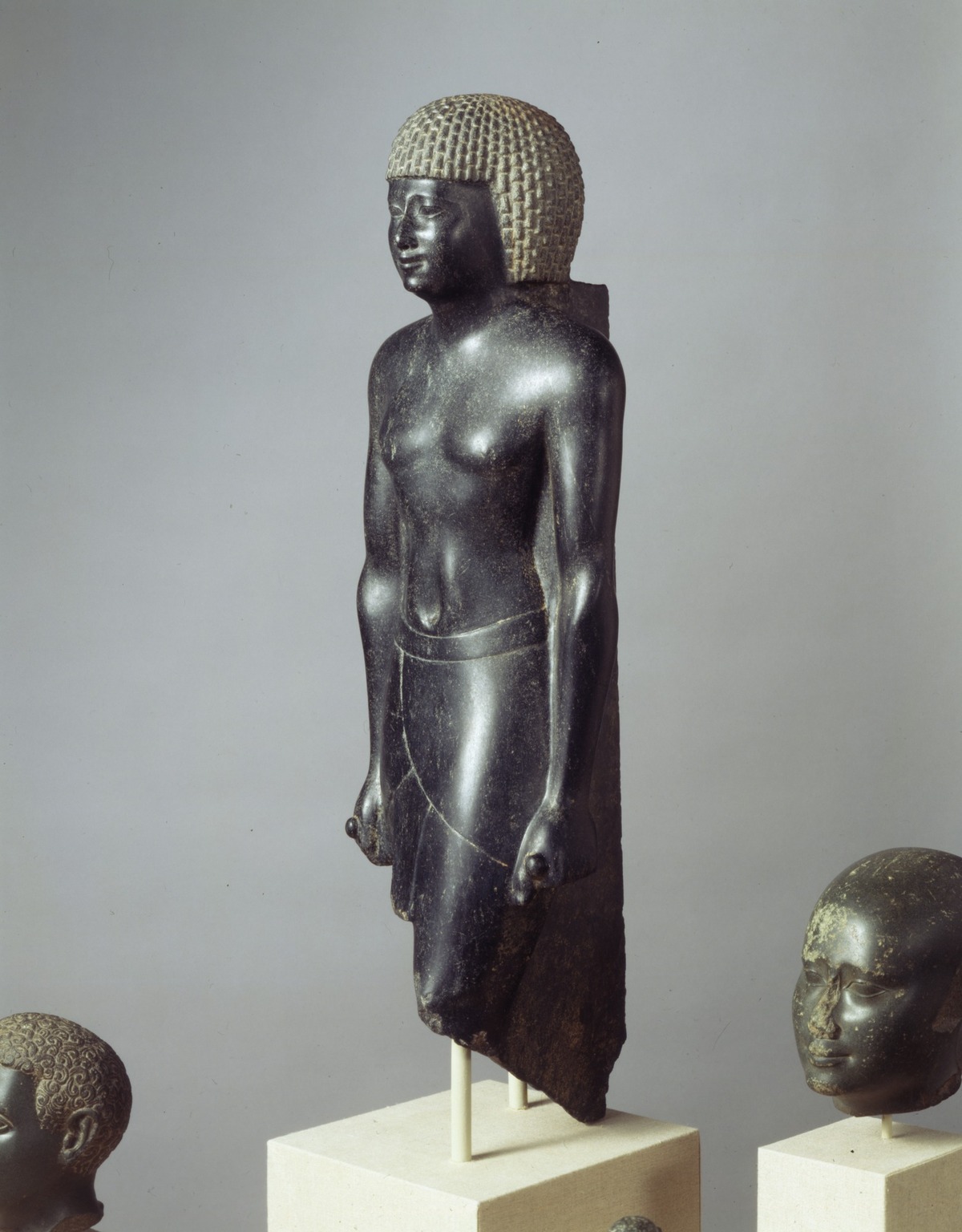The photograph, taken in a museum with a dark gray background, features a central statue flanked by two smaller sculptures, all exhibited on white stands. The main statue in the center portrays a woman with golden hair, rendered in shiny black stone. She appears to be wearing a headpiece and a long skirt, but her legs are missing, leaving only the upper body and dress visible. This central figure faces towards the left side. On the bottom left, a partially visible black stone head, presumably with short curly golden hair, accompanies the main statue. To the bottom right, another black stone head is displayed; it is more worn and lacks hair. All the sculptures exude an archaeological or possibly Egyptian cultural ambiance with their distinct features and craftsmanship.